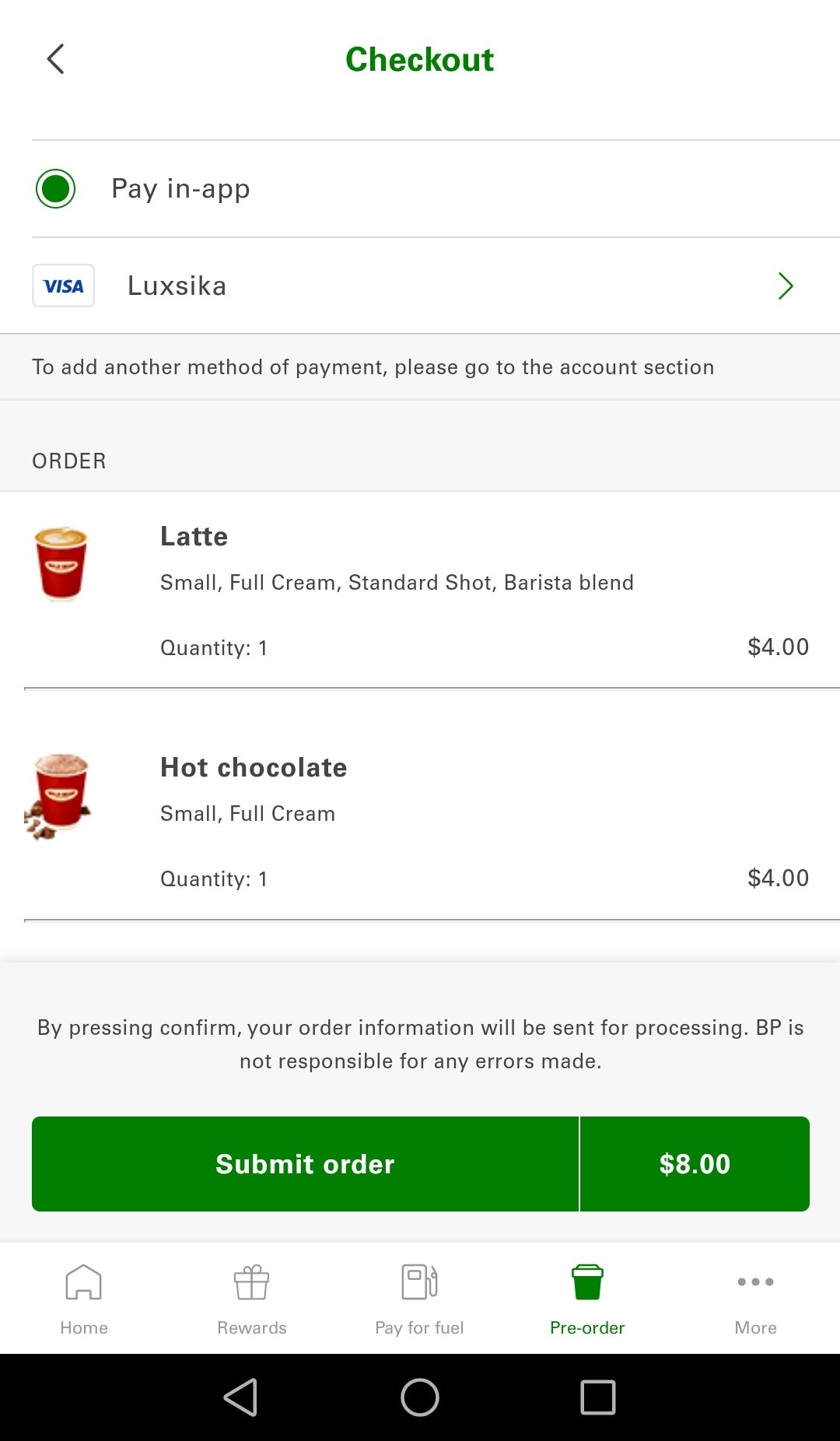In the image, there is an interface displaying a checkout process. To the left, an arrow points to the "Checkout" button, which is highlighted in green. Various payment options are listed, including Visa and Lux Sikca, with a prompt to add another payment method through the account section. An order summary shows the details of two items: a small latte with full cream and a standard shot made with Brewster blend, priced at $4, and a small hot chocolate with full cream, also priced at $4, totaling $8. Below the summary, instructions indicate that by pressing "Confirm," the order information will be sent for processing, with a disclaimer stating that BP is not responsible for any errors. 

The screen also features a green rectangle labeled "System Order" with the total amount displayed as $8. Navigation buttons include a home button, a rewards button, a button to pay for fuel, a pre-order button, and an ellipsis for additional options. A black rectangle at the bottom contains a left arrow, a circle, and a square, suggesting control or action buttons. Additional decorative lines are also present on the interface.